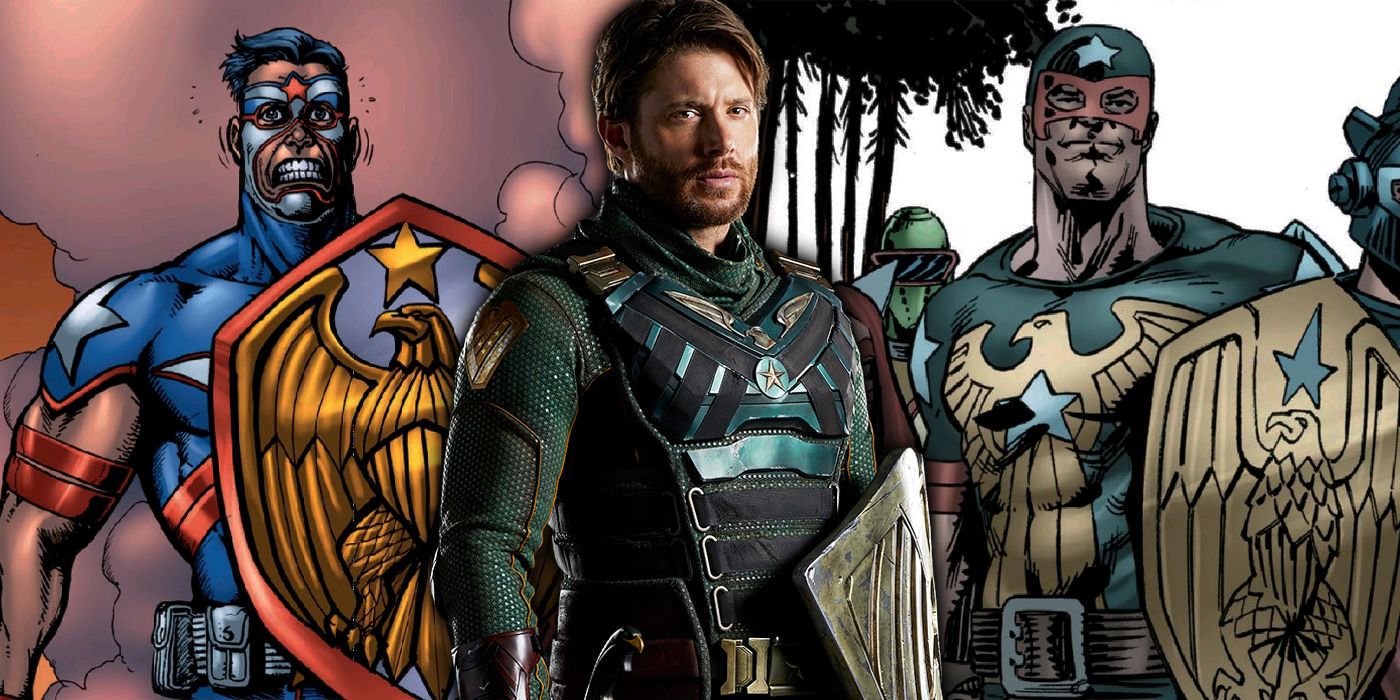The image features a central character, a live actor dressed in an emerald green and black superhero suit accented with gold. The actor, who has long brown hair, a full beard, and an intense expression, wears a V symbol crisscrossed with an American flag pattern on his shoulder. He is holding a shield, though its details are partially obscured. Flanking the actor on both sides are illustrations of similar superhero characters. The left illustration shows a character in red, white, and blue American-themed gear, equipped with a shield displaying a gold eagle and a star above it. The right illustration depicts another superhero in a similar color scheme, also adorned with a gold eagle on his chest and holding an all-gold shield with an eagle emblem. Both illustrated characters wear tight shirts, and the motifs they bear closely resemble the central live-action character's design.